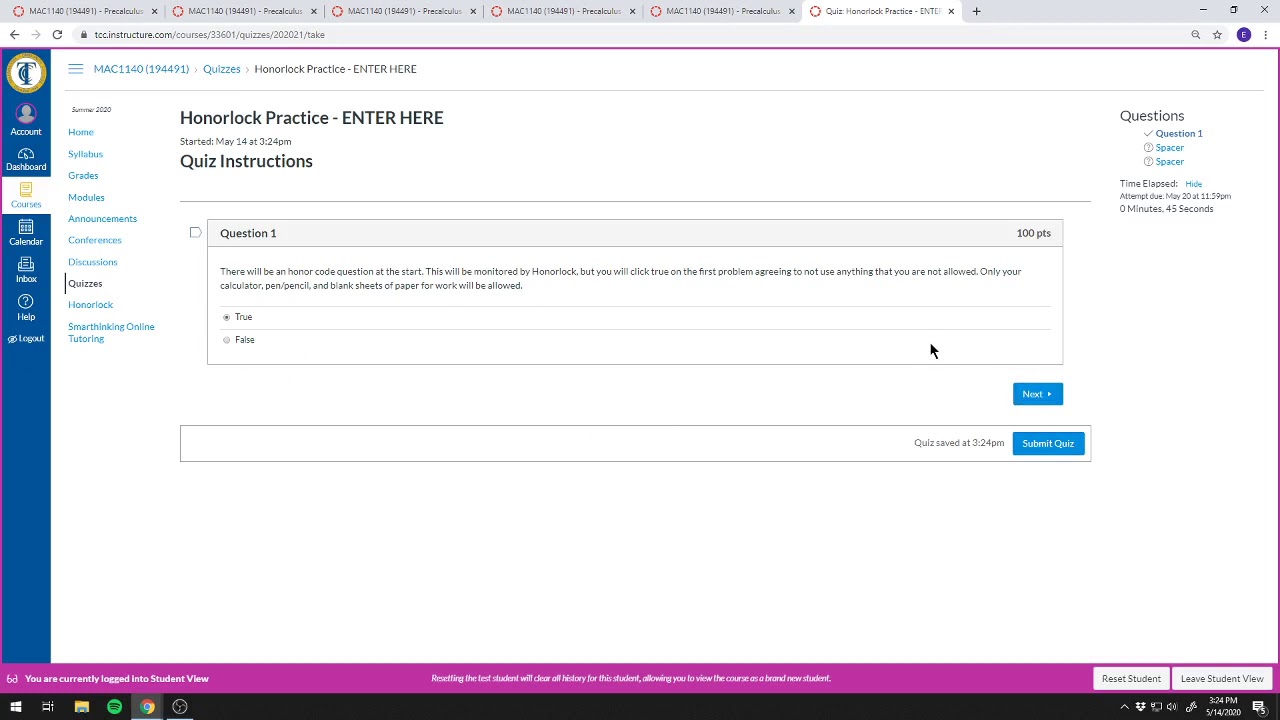The image displays a screenshot of a web page viewed in a Google Chrome browser. There are six tabs open, with the sixth tab currently active. In the upper right corner, standard window control icons are visible: options to minimize, maximize, or close the window. The browser’s bottom bar is black, displaying various icons including the Windows logo, a file icon, the Spotify logo, the Chrome logo (selected), and another indistinguishable logo. The far right of this bar features more icons and displays the current time as 3:24 PM.

Below the browser tabs, there are standard navigation icons: back, forward, refresh, and a lock icon, alongside an unreadable website address. 

The web page itself has a blue sidebar on the left with several labeled icons. At the top is a yellow-rimmed circle with a white center and a blue "T". Below it, an icon depicts a silhouette labeled "Account". Further down, a cloud icon labeled "Dashboard", a file icon labeled "Courses", a calendar icon labeled "Calendar", a paper icon labeled "Inbox", a question mark icon labeled "Help", and finally, "Logout".

To the right of the sidebar, the top section of the page contains three horizontal lines, a label "Mac 1140 (194491)", and further sections labeled "Quizzes", "Honor Lock", and "Practice". Below a gray line, another column links to "Summer something", "Home", "Syllabus", "Grades", "Modules", "Announcement", "Conferences", "Discussion", "Quizzes", "Honor Lock", and "Smart Thinking Online Tutoring", with "Quizzes" currently selected.

The main content area presents details for the “Honor Lock Practice” quiz. It started on May 14th at 3:24 PM, under the heading "Quiz Instructions". Following another gray line, "Question 1" is worth 100 points. The question text, although unreadable, involves agreeing to an Honor Code by selecting "True" or "False." "True" is chosen and a blue "Next" button is available below. Another timestamp shows "Quiz Saved at 3:24 PM", and a "Submit Quiz" button is visible.

On the far right, a section lists quiz navigation elements, including "Questions" with checkmarks and time-related data: "Question 1," placeholders for additional questions, "time elapsed," and an "attempt due May 20th, 11:59 PM", with currently "0 minutes and 45 seconds" elapsed.